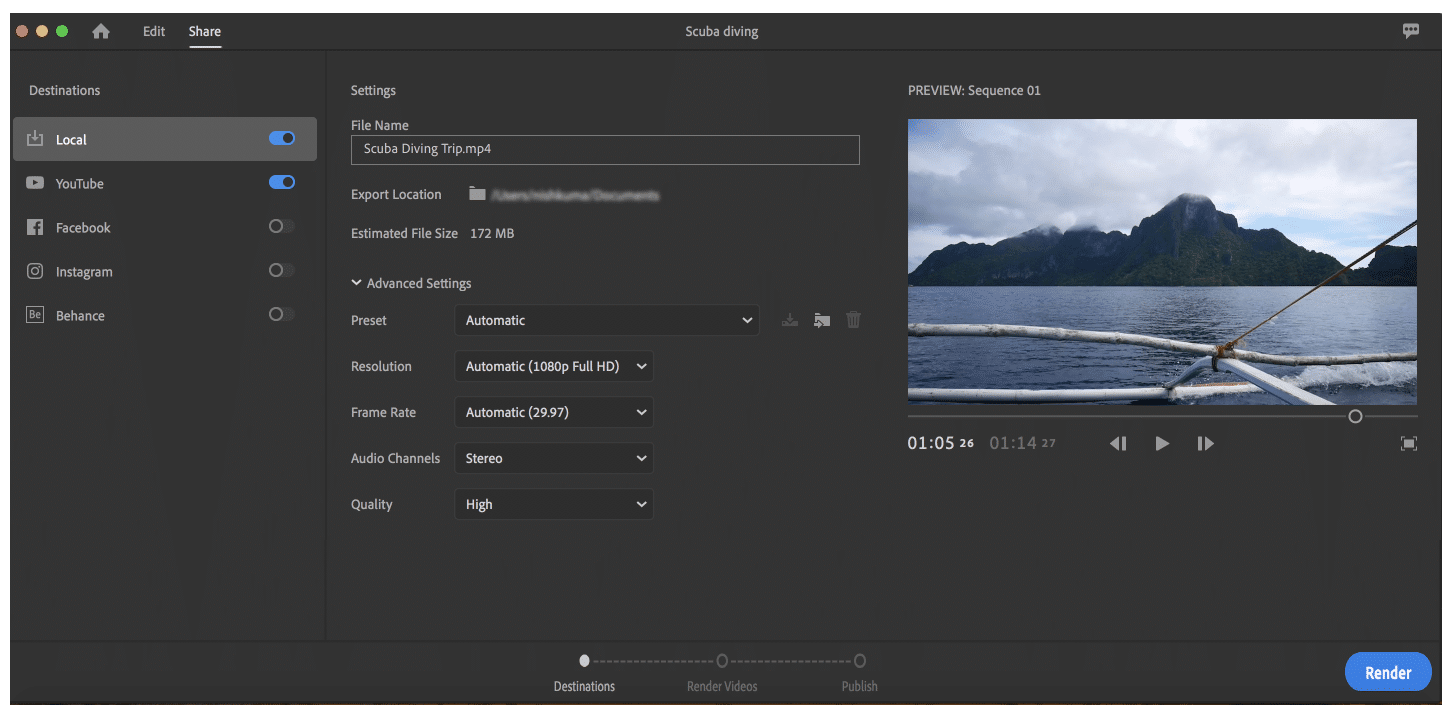In this image, set on a Mac device, the top left corner features three small circles: the first in brown, the second in pink, and the third in green. To the right of these circles, there is a house icon. Further to the right, the words "Edit" and "Share" are displayed, with "Share" highlighted in bright white and underlined. Centered at the top, the text "Scuba Diving" is visible. The top right corner contains a chat bubble icon.

In the middle section of the image, positioned to the right, there is a paused video within a square frame. The video captures a scene of boating on a large body of water, with a towering mountain and overhead clouds in the background. 

In the center of the image, there are several settings displayed. The term "File Name" is followed by a text box labeled "scubadivingtrip.mp4." Below this, "Export Location" and "Estimated File Size 172 MB" are indicated. In the bottom right corner, a small circular button labeled "Render" is visible.

On the left side of the image, the word "Destinations" appears, with several categories listed below, including Local, YouTube, Facebook, and Instagram.